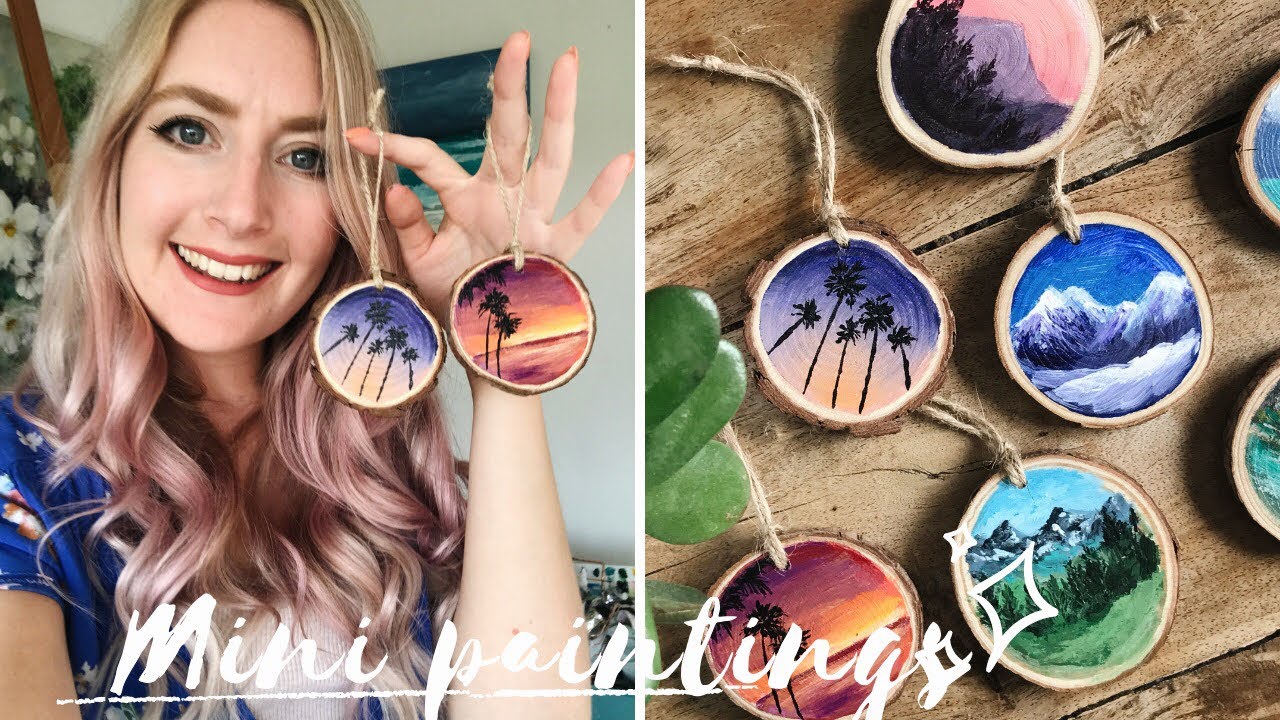A blonde white woman with blue eyes is smiling warmly while showcasing her handmade mini paintings. She is dressed in a blue shirt or dress with a print, and her hair transitions from blonde at the top to a pinkish blonde at the bottom. She is holding up two of her mini paintings on her left hand, dangling them from strings looped around her forefinger and middle finger, palm facing forward. The paintings are crafted on thin, bark-framed slices of wood, each depicting serene landscapes. One artwork features palm trees under a bright blue sky, while another captures a sunset over a beach. Additional pieces illustrate snowy mountains, green mountainous landscapes, and forested hills with rocky outcrops reminiscent of the Blue Ridge Mountains. The images have a modern aesthetic, and the words "mini paintings" are visible at the bottom of the photograph, suggesting it could be an advertisement for her art.